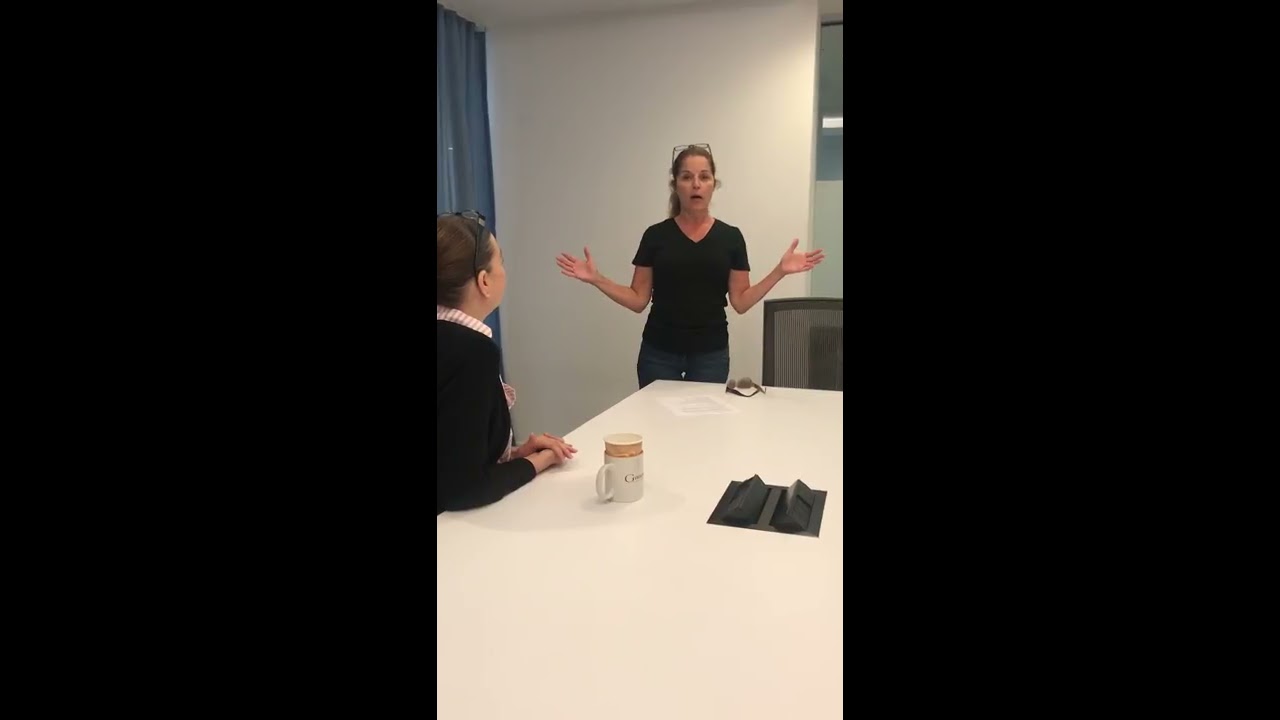In an indoor office setting, two Caucasian women with brown hair and glasses perched on top of their heads are depicted in a detailed scene. On the left side of the image, a woman is seated at a white table, wearing a black jacket over a striped tan and white shirt. Her hands are folded in front of her, and a mug with a paper cup inside sits beside her. She listens attentively to the standing woman on the right, who is presenting with her hands outstretched and elbows at her sides. This woman wears a black V-neck shirt and blue jeans, and has a pair of sunglasses resting on the table near a black mesh chair beside her. The table features a black box with pop-up plug outlets in its center. Blue, floor-to-ceiling curtains flank the seated woman on the left, completing the room’s decor.